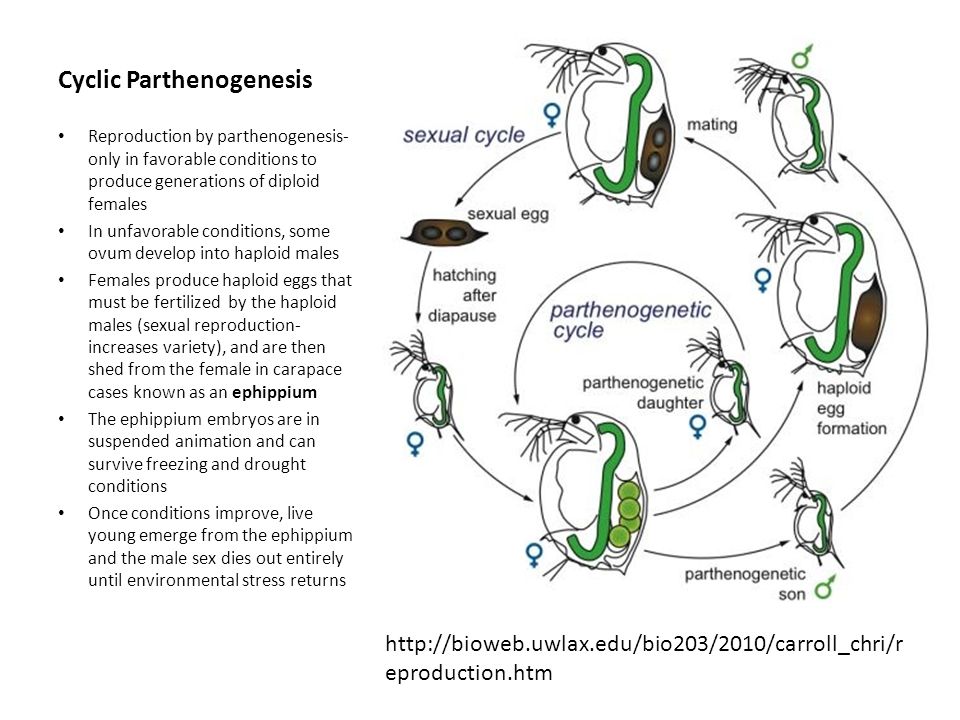The image is a detailed diagram illustrating the process of cyclic parthenogenesis, prominently titled in bold at the top left. It includes a series of drawings and text descriptions that explain this complex reproductive cycle. The diagram begins with a bulbous, insect-like creature, which features an antenna and is depicted at the bottom with a tube holding green eggs. Arrows connect different stages of the cycle, showing transitions from parthenogenetic sons and daughters to haploid egg formation and subsequent mating.

The cycle described involves reproduction by parthenogenesis during favorable conditions, producing generations of diploid females. Under unfavorable conditions, some develop into haploid males. Females produce haploid eggs that must be fertilized by these males, and sexual reproduction enhances genetic variety. The fertilized eggs, encased in a structure called epifibium, enter a state of suspended animation, capable of surviving extreme conditions like freezing and drought. When conditions improve, the embryos hatch, emerging as live young, and the male population dies out until environmental stress triggers the cycle again.

Further bullet points on the left elaborates on these stages. The right side of the diagram visually represents the transitions: starting from sexual egg to sexual cycle, mating, haploid egg formation, and then to parthenogenetic offspring. The creatures in the diagrams resemble bird-like figures despite the insect context, adding to the illustrative detail.

Additionally, the image notes a reference website, http://bioweb.uwlax.edu, at the bottom for further information.